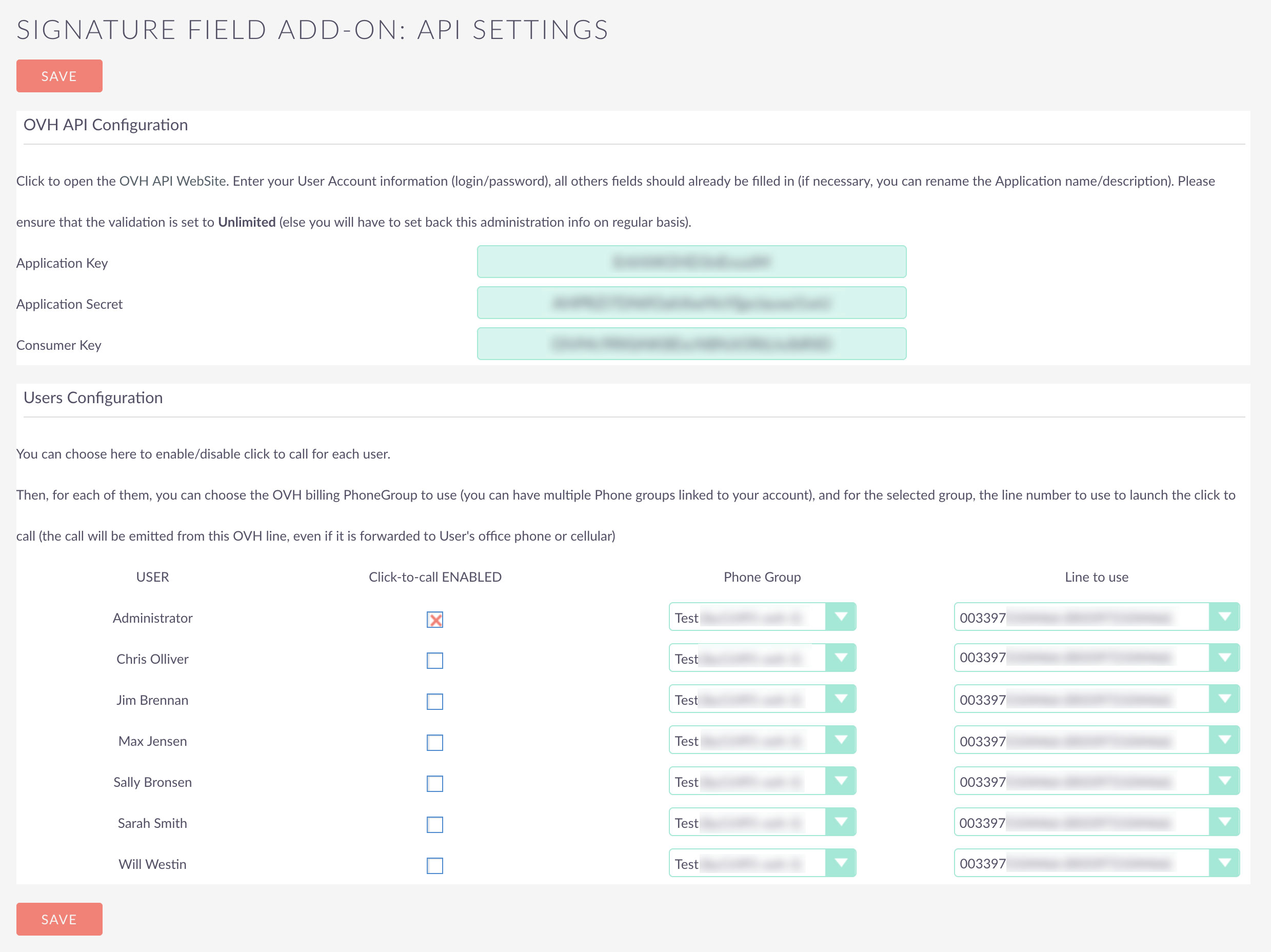The image is a screenshot of a settings or configuration webpage. At the top, the heading reads "Signature Field Add-On." Beneath this heading, a peach-colored "Save" button is prominently displayed. Below the button, the section titled "OVH API Configuration" is visible. This section instructs the user to "Click to open the OVH API website" and prompts them to enter their user account information, including login and password. It notes that all other fields should already be filled in. Additionally, it advises users that the application's name/description can be renamed and prompts them to ensure that the validation is set to "unlimited" to avoid having to reenter the administration info regularly.

In this section, the fields for "Application Key," "Application Secret," and "Consumer Key" are all blurred out for privacy. Further down, another section labeled "User Configuration" is visible, where users have the option to enable or disable the "Click to Call" feature for each individual user. Similar to the previous section, most of the fields here are also blurred out.